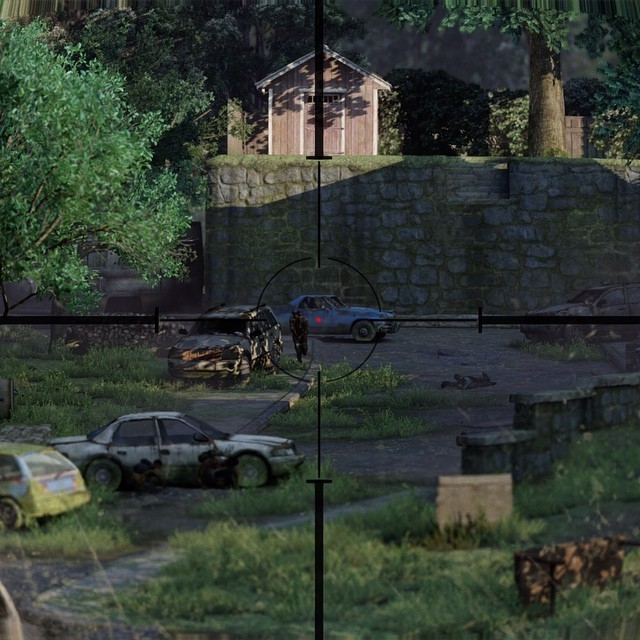The image appears to be a highly realistic screenshot from a video game showcasing an outdoor scene, reminiscent of a post-apocalyptic world. The square-shaped scene is filled with dark green grass, abundant vegetation, and multiple damaged cars, giving it an abandoned parking lot ambiance. The terrain includes a little valley with various wrecked vehicles, such as a yellow damaged car, two white burnt-out cars, and a blue car, all surrounded by overgrown grass.

In the background, there's a tall stone wall, approximately 10 to 15 feet high, crowned with grass and a small red shed with white trim. The overabundance of unkempt foliage throughout the image suggests a setting where nature is reclaiming the environment due to the absence of human maintenance.

At the center of the image is a black-clad soldier, seen from a first-person perspective, running close to a red crosshair superimposed on the screen. The crosshair, featuring a red dot in the middle, indicates that the player is aiming a gun at the soldier, emphasizing the combat scenario typically found in video games.